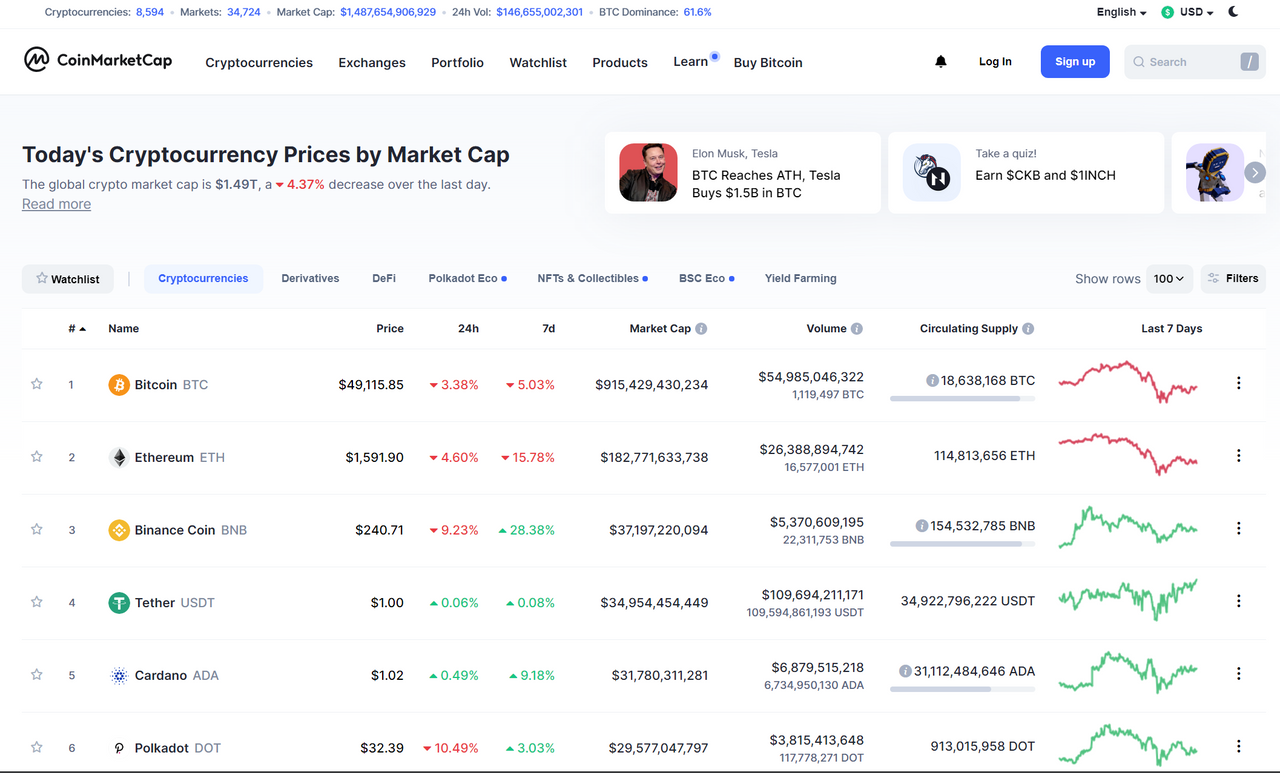This detailed caption provides a vivid description of the screenshot of the web page showing cryptocurrency information:

"The screenshot depicts a web page from CoinMarketCap with comprehensive cryptocurrency details. The top section of the page features a clean white background serving as a header, while the lower section transitions to a gray background. A thin black line runs horizontally across the bottom of the screenshot, providing a clear separation.

In the top-left corner, there is a horizontal information bar displaying vital statistics: 'Cryptocurrencies: 8,594', 'Markets: 34,724', 'Market Cap: $1,487,654,906,929', '24-Hour Volume: $146,655,002,301', and 'BTC Dominance: 61.6%'. 

The upper right corner of the header includes a drop-down menu for language set to English, and another for currency set to USD, accompanied by a crescent moon logo indicating a theme or display option. Below this, the CoinMarketCap logo is prominently placed with the text 'CoinMarketCap' beside it.

Directly beneath the logo is a navigation menu with options for 'Cryptocurrencies', 'Exchanges', 'Portfolio', 'Watchlist', 'Products', 'Learn', and 'Buy Bitcoin'. A small blue dot is visible atop the 'Learn' option, possibly indicating a new feature or notification.

Towards the right side of the header, there is a bell icon for notifications, followed by buttons for 'Login' and 'Sign Up', and a search bar for easy navigation."